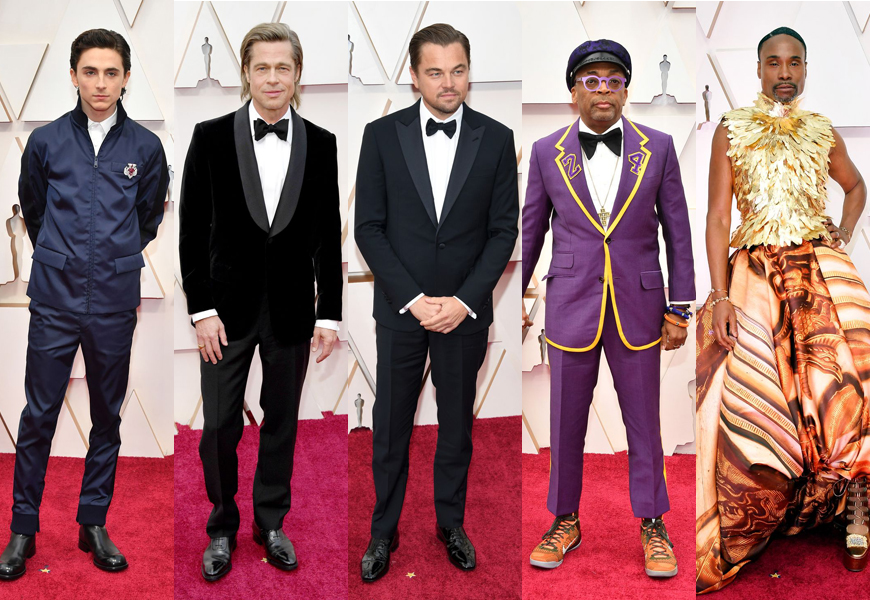The image is a composite of five narrow, vertical rectangular photos, each showcasing different actors standing on a red carpet with a white background. From left to right, the first actor is Timothée Chalamet, dressed in a navy blue suit with a white collared shirt, black boots, and sporting short brown hair. Next is Brad Pitt, who is wearing a classic black tuxedo with a white shirt, black shoes, and has brown hair. Following him is Leonardo DiCaprio, adorned in a black and white tuxedo, with brown hair and black shoes. The fourth individual is Spike Lee, recognizable in a vibrant purple suit with yellow trim and purple glasses. His outfit also features a number 24, paying tribute to Kobe Bryant, and a white shirt with a black bowtie. Lastly is Billy Porter, an African-American actor, wearing a standout outfit consisting of a glittery, sleeveless gold top paired with a patterned skirt in shades of tan, brown, and dark brown. His ensemble is complemented by a vest resembling eagle's fur and a bracelet. The cohesive background of the red carpet ties all these distinct fashion statements together.